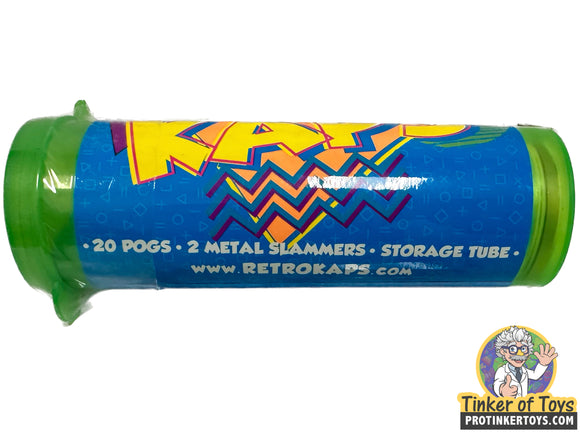This image showcases a modern remake of a classic toy from Tinker of Toys, now branded as Retro Caps. The toy consists of a vibrant lime green plastic tube with a flip-top cap, photographed horizontally against a white background. This sleek storage tube is decorated with a dark blue label featuring a playful design of geometric shapes, such as circles, triangles, diamonds, and mathematical symbols. Prominently displayed in yellow bubble letters is the word "CAPS," partially visible and horizontally stretched across the label, with purple jagged squiggles beneath it. The label provides essential details in white text, indicating the contents: "20 POGs, 2 metal slammers, storage tube," and directs viewers to visit www.retrocaps.com for additional information. Additionally, the Tinker of Toys logo, showcasing a quirky scientist with gray hair, glasses, and a mustache, donned in a white coat and set against a green and purple bubble background, is prominently featured. Accompanying the logo is the web address protinkertoys.com, providing a nod to the toy's nostalgic roots.